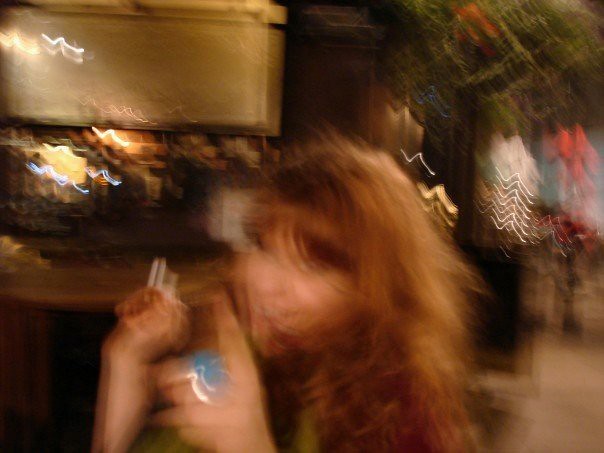This photograph, though blurred due to evident motion during capture, reveals a scene set in what seems to be an illuminated room, possibly a bar. Dominating the image's center is a woman, presented from just below her elbows upward. Her light-skinned face, framed by long red hair and bangs, faces forward slightly angled to the right. She appears in an ambiance suffused with warm light and visible fixtures. Above her, toward the top of the frame, is a distinctive gold rectangle. In her right hand, she delicately holds a cigarette, while her left hand clutches an unidentified blue object or possibly wears a blue ring. The background, particularly beneath the golden rectangle, hints at a bar setting with numerous lights and the hazy outlines of bottles, adding to the image’s atmospheric depth.